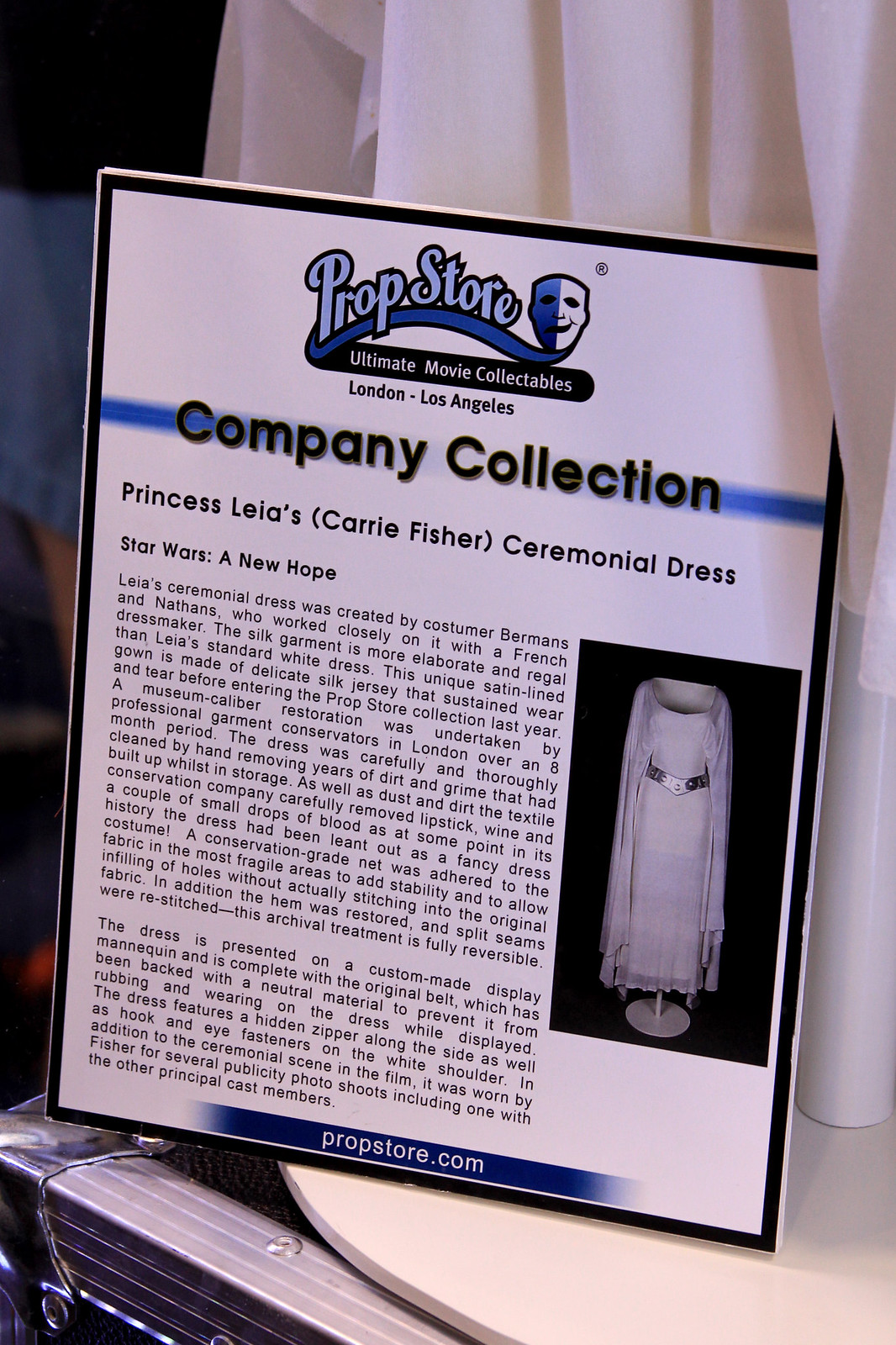This full-color photograph captures a detailed informational plaque from the Prop Store, known for its ultimate movie collectibles, based in London and Los Angeles. The rectangular plaque, bordered in black, is presented on white paper and features a combination of blue and black text. At the top, it reads "Prop Store, Ultimate Movie Collectibles,” followed by “London, Los Angeles, Company Collection.” The main section identifies the item as “Princess Leia's (Carrie Fisher’s) ceremonial dress from 'Star Wars: A New Hope'.” The informative text below elaborates that this is the iconic dress worn by Princess Leia during the medal ceremony scene at the end of the movie, where she awards Han Solo and Luke Skywalker for their bravery in destroying the Death Star. A detailed photograph of the dress is positioned on the right side of the plaque, showcasing the white gown with long sleeves, a cloak-like cape, and a silver belt. The background of the image hints at the actual dress displayed on a white base. The plaque also mentions that Carrie Fisher wore this dress for several publicity photo shoots, including those with other principal cast members. At the bottom of the plaque, a blue banner with white text reads "PropStore.com."